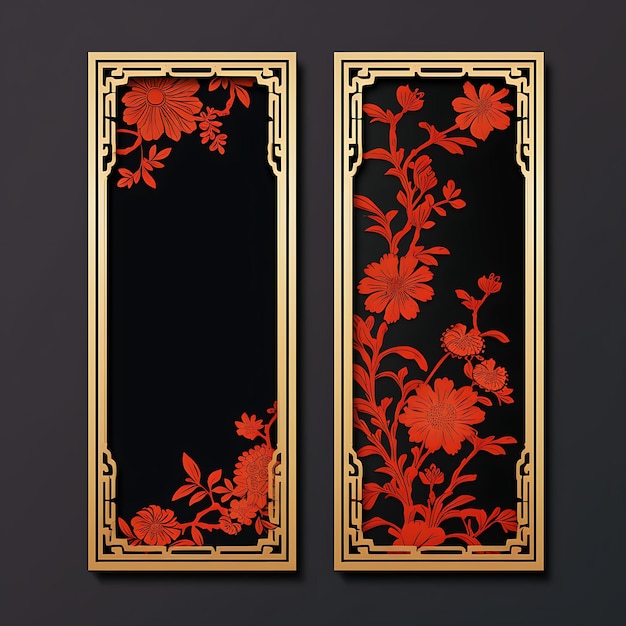The image showcases two rectangular framed artworks placed side by side against a dark grey background. Each frame is adorned with intricate golden borders, featuring dual parallel stripes along the edges and elaborate linear designs at the corners. Both frames have black backgrounds but differ in the arrangement of their floral patterns. The frame on the left displays vivid red flowers positioned at the top left and bottom right corners, leaving the center as an empty, pitch-black space. In contrast, the frame on the right is dominated by a curving floral stem that grows from the bottom left and extends to the top, filled with flowers and leaves that cover most of the black background.